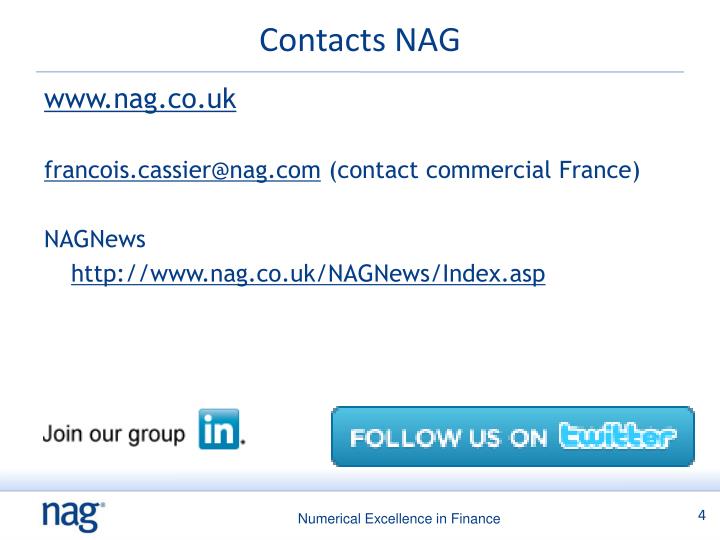The image is a text-heavy screenshot with blue lettering on a white background, resembling an online advertisement. At the top, in bold print, it reads "Contacts NAG," followed by a pale blue line underneath. Below this line is the web address "www.nag.co.uk" in dark blue, underlined. Underneath it is the email "francois.cassier@nag.com," accompanied by the parenthetical note "(Contact Commercial France)." 

Further down, another bold blue line reads "nagnews," beneath which is a web address "http://www.nag.co.uk/nagnews/index.asp," also underlined. At the bottom of the ad, it says "Join Our Group" in black text, next to a blue box labeled "IN," indicating a LinkedIn logo, followed by a banner stating, "Follow us on Twitter." Additional text along the bottom includes "nag" on the left, "Numerical Excellence in Finance" in the center, and the number "4" on the right.